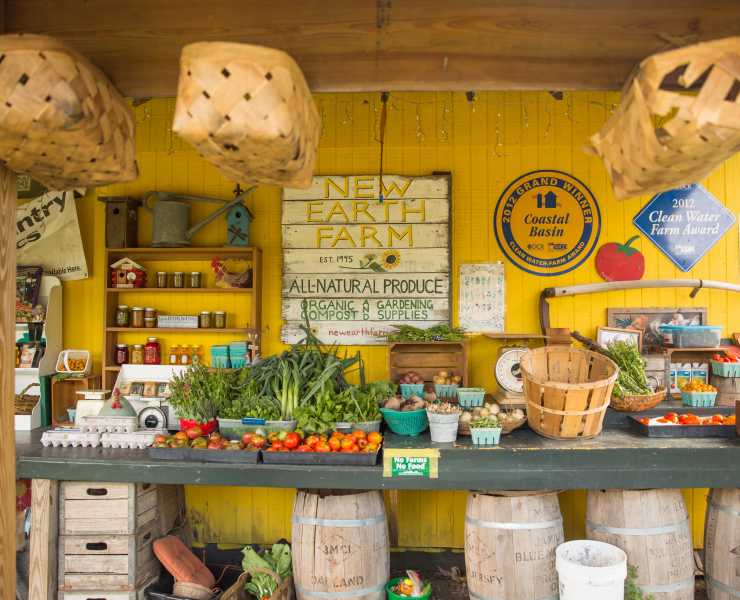The photograph captures a vibrant farm produce stall with a bright yellow-painted wooden background and a wooden roof overhead. Centered on the wall is a prominent sign painted on barn wood, announcing "New Earth Farm, Established 1995" in bold yellow and green letters. Beneath the farm's name is a painted sunflower and the text "All Natural Produce, Organic Compost, and Gardening Supplies." To the right of this main sign are two notable awards: a circular yellow and blue sign proclaiming "2012 Grand Winner Coastal Basin" and a blue diamond-shaped sign declaring the "2012 Clean Water Farm Award."

Suspended from the ceiling are three wicker baskets, adding to the rustic charm. Below, a dark green wooden table stands out, with four beige barrels on its right side and three stacked wooden crates on the left. Between these, various baskets and buckets brim with green leaves and an orange, pillow-like object. Atop the table, on the left side, are three stacked egg cartons, followed by black bins overflowing with red and green tomatoes. Further right, there are clear plastic bins containing an assortment of green vegetables.

Continuing along the table, a variety of blue and white containers hold round, brown objects, possibly small potatoes. Nearby, a wooden basket sits in front of a scale, while an array of baskets filled with green and orange vegetables complete the display. The setup conveys a busy yet organized farm stand, offering an assortment of fresh produce, including tomatoes, onions, garlic, and jams and jellies on a rear shelf. The overall effect is a lively and inviting snapshot of farm life and local goods.